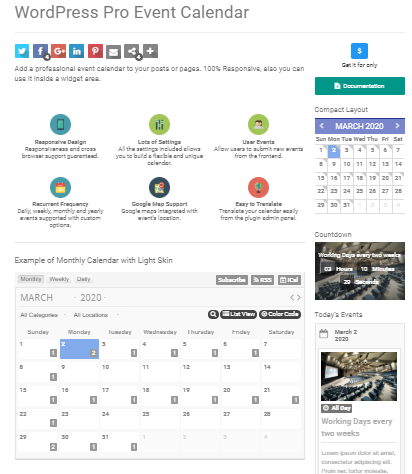Screenshot of a Webpage Featuring WordPress Pro Event Calendar Plugin

The image captures a webpage showcasing the WordPress Pro Event Calendar plugin. At the top left of the screenshot, the title "WordPress Pro Event Calendar" is prominently displayed in a grayish-black color with each word capitalized. Directly beneath the title is a thin gray line extending across the width of the page.

Under this line, on the left side, there are several small icon squares that correspond to various social media platforms and actions, such as Tweet, Facebook, Google, LinkedIn (N), Pinterest, Mail, Merge, and Plus.

The main body of the page features a section promoting the key features of the calendar plugin. The description highlights that the calendar can be added to posts or pages and is 100% responsive, also stating that it can be used within a widget area.

Below this, there are two rows of feature icons:

- **First Row (from left to right)**:
  1. A blue circle with a phone icon, indicating "Responsive Design."
  2. A green circle with a settings icon, labeled "Lots of Settings."
  3. Another green circle with a user icon, representing "User Events."

- **Second Row (from left to right)**:
  1. A blue circle containing a yellow and red symbol, labeled "Recurrent Frequency."
  2. A black circle with a map icon, indicating "Google Map Support."
  3. A red circle with a globe icon, representing "Easy to Translate."

Beneath these icons is another gray line followed by a preview of a monthly calendar with a light skin theme, displaying March 2020. At the top of this calendar view, users can choose to display the calendar in "Monthly," "Weekly," or "Daily" formats. To the right, three tabs labeled "Subscribe," "RSS," and "iCal" are visible.

Additional options include a search bar, listing view, color guide, and customizable calendar features. To the right of the calendar, a blue box indicates a pricing detail with a label "Get it for only $" followed by a green bar titled "Documentation."

A compact layout is shown, featuring a small calendar for March 2020 with a blue header. It includes functionalities such as displaying calendar pages, showing countdowns, and tracking working days. The current day’s events, hours, minutes, and seconds are also presented, providing a comprehensive view of the plugin’s customizable document capabilities.